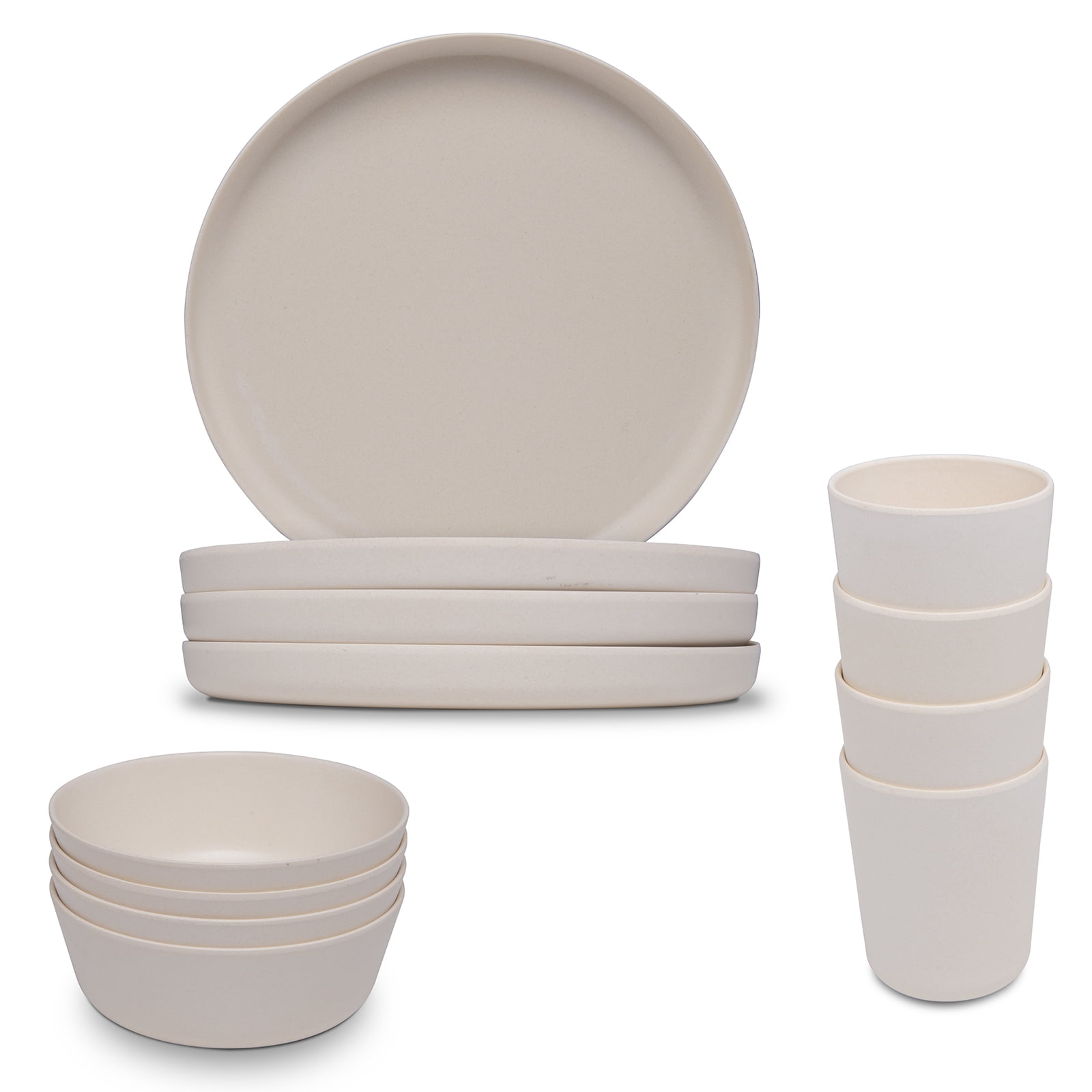The image is a detailed photograph of an assortment of white ceramic dinnerware, featuring plates, bowls, and cups, all stacked in distinct sets against a white background. Positioned upright at the top right of the image is one flat plate, accompanied by three more lying flat. Below and to the left, four shallow bowls are stacked neatly, each mirroring the flat plates in their white eggshell color and ceramic material. To the lower right, a similar arrangement holds four cups, which share the same material and color as the plates and bowls. The minimalist setup showcases the simplistic yet elegant design of the dinnerware, though opinions on its aesthetic appeal vary. Overall, the photograph highlights the cohesive nature of the three sets of containers, emphasizing their uniform color and material.